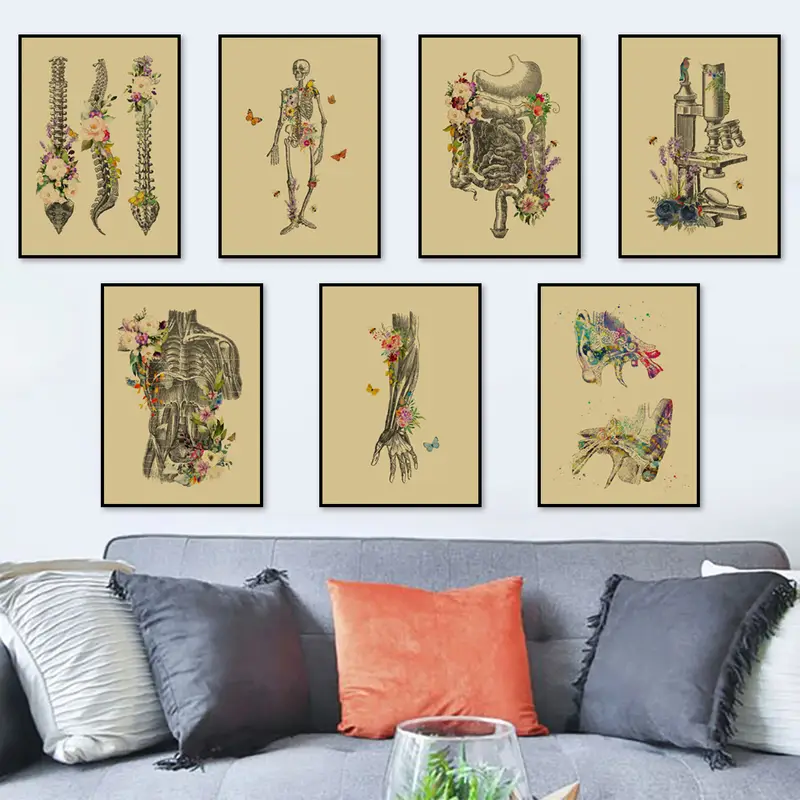The photograph depicts a living room with a vertical rectangular layout. Dominating the center is a stylish blue couch adorned with five distinct throw pillows. Centrally placed is a striking orange pillow, flanked on either side by gray pillows in varying shades—dark gray to the left and light gray to the right. Additionally, there is a solid blue pillow with fringes and a striped white pillow.

In front of the couch, a glass terrarium serves as a table centerpiece, showcasing thriving green plants within.

Above the couch, seven meticulously arranged paintings draw the eye. These anatomical artworks, each set against a brown background and framed in black, are displayed in two rows: four evenly spaced on the top row and three staggered directly below. The top row features an intricate spine with plants, a full skeleton adorned with flowers or butterflies, the digestive system interwoven with flora, and a microscope with floral elements. The bottom row continues the theme with the muscular system, arm muscles, and anatomical details of the ears, all depicted with flourishing botanicals.